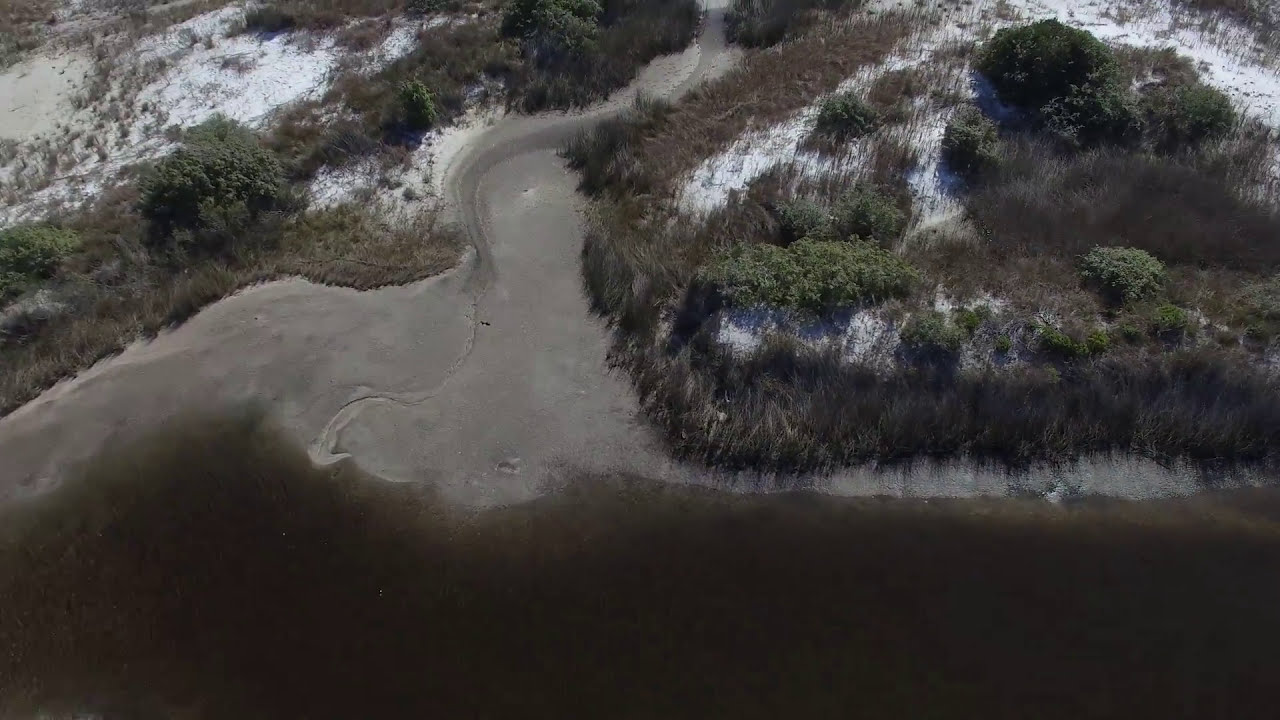This aerial daylight photograph captures a natural landscape, predominantly showcasing a dried, curving riverbed that appears brown or green, likely due to underlying moss or reflections. The bottom of the image features dark brown, almost muddy water that is opaque and could be shallow, with visible underwater vegetation. Surrounding this dried riverbed is a gradient of ground colors: brown, covered with dried grass closer to the shore, and transitioning to a snowy or exceptionally white sandy terrain further away. The land rises on both sides of the riverbed, with areas covered in short brown grass, green shrubs, and scattered trees. The scene suggests a mixture of seasons, with green vegetation standing in stark contrast to the snow or white ground, indicating a dynamic and diverse ecosystem. The image also hints at a wash embankment on the left, possibly formed by rainwater runoff from nearby mountains, integrating elements of both winter and a broader natural water drainage system.